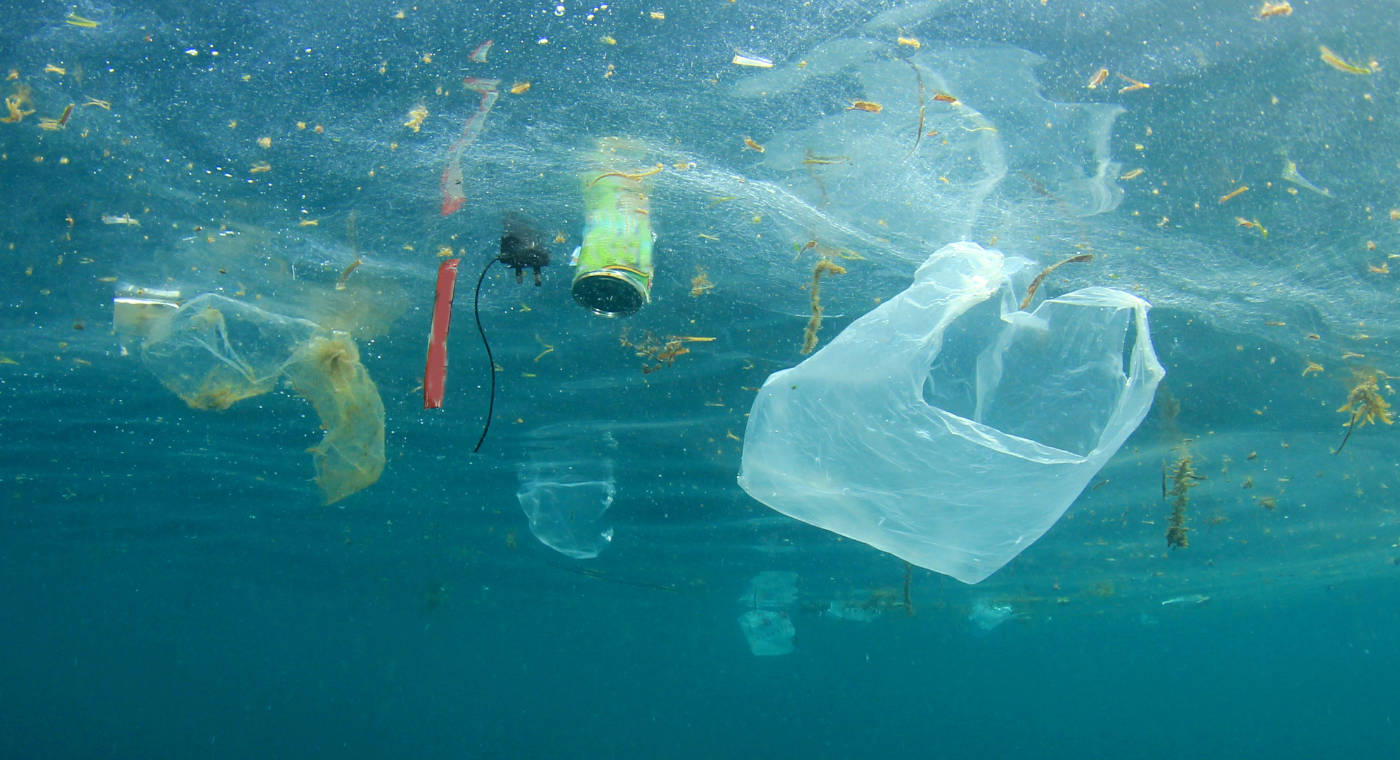The image depicts an underwater scene viewed from a couple of feet below the surface in what appears to be the ocean or a lake. The water transitions from a teal color at the bottom to a light blue near the surface, where an array of floating trash is visible. Prominently in the foreground is a somewhat transparent white plastic bag. A green can with a silver bottom hangs down, accompanied by a black piece of plastic with a long black line and a red board-like object hanging almost straight down. Surrounding this area is floating green moss, contributing to the murky appearance.

Further to the left, a plastic piece encased in green algae resembles a jellyfish. Scattered around the area are additional items of litter, including another clear bag with brown debris, various other clear bags in the background, and a plastic bottle with some kind of film on it. Among the debris is a black electrical cord with a plug. White bubbles populate the water's surface, emphasizing the contrast between the cleaner bottom and the trash-laden top. The overall scene highlights the ecological impact of litter and conveys a strong message about pollution and the environment.